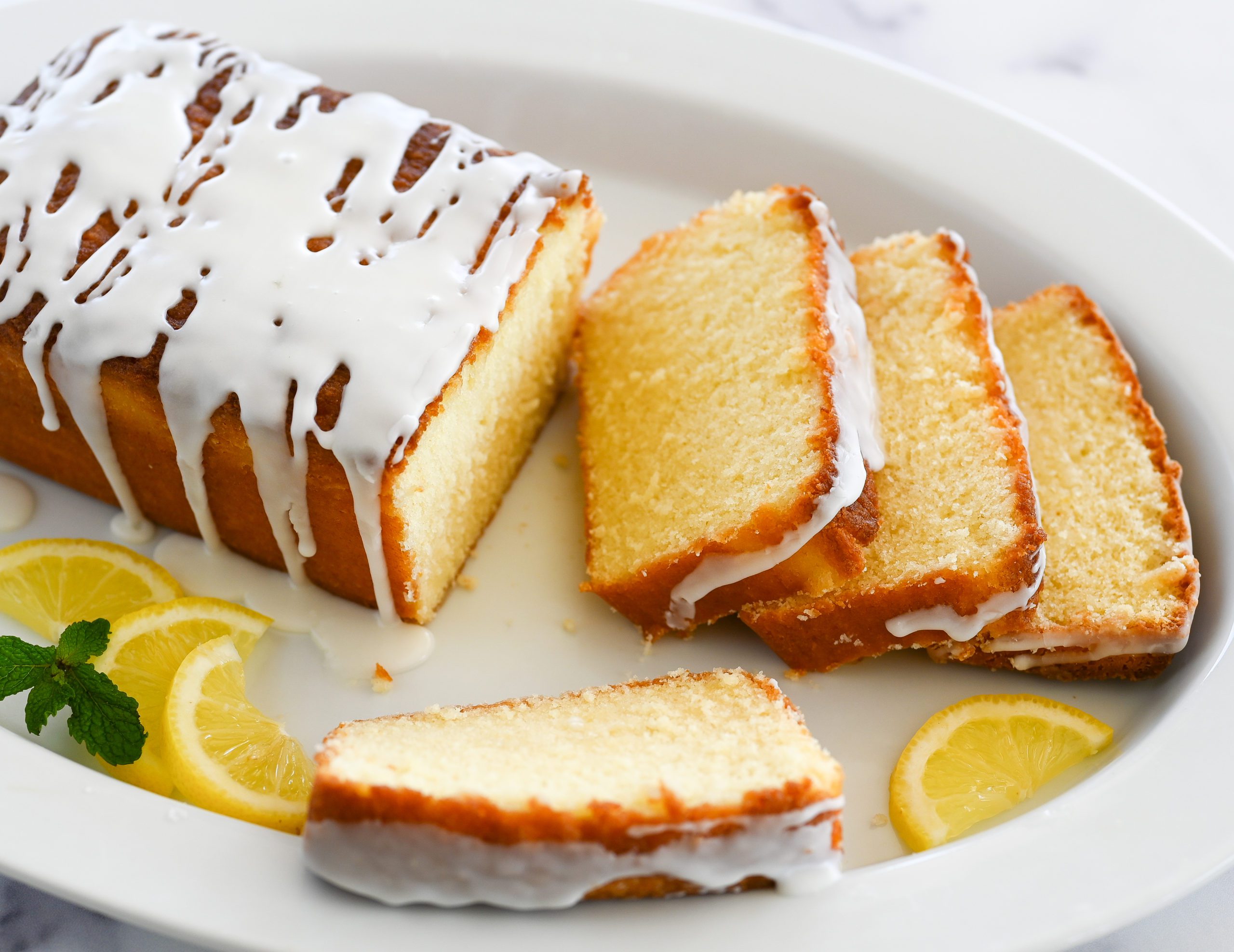This is an overhead, slightly angled photograph of a white dish set on a marble countertop. The dish, which resembles a large bowl platter, contains a pound cake divided into five sections. The left side holds the majority of the cake, which is uncut, while the other four sections are individual slices. The cake features a yellow interior and a brown crust, with a white sweet glaze drizzled over the top, pooling at the bottom of the dish. Three of the slices are overlapping each other near the top right, and another slice leans against the edge at the bottom. Surrounding the cake are accoutrements, including four lemon slices, some scattered near the base of the cake and one at the front bottom right of the dish, along with a piece of green garnish or parsley for decoration. The background is predominantly white with gray specks visible in the upper corners. The composition and meticulous details suggest a professional quality image.